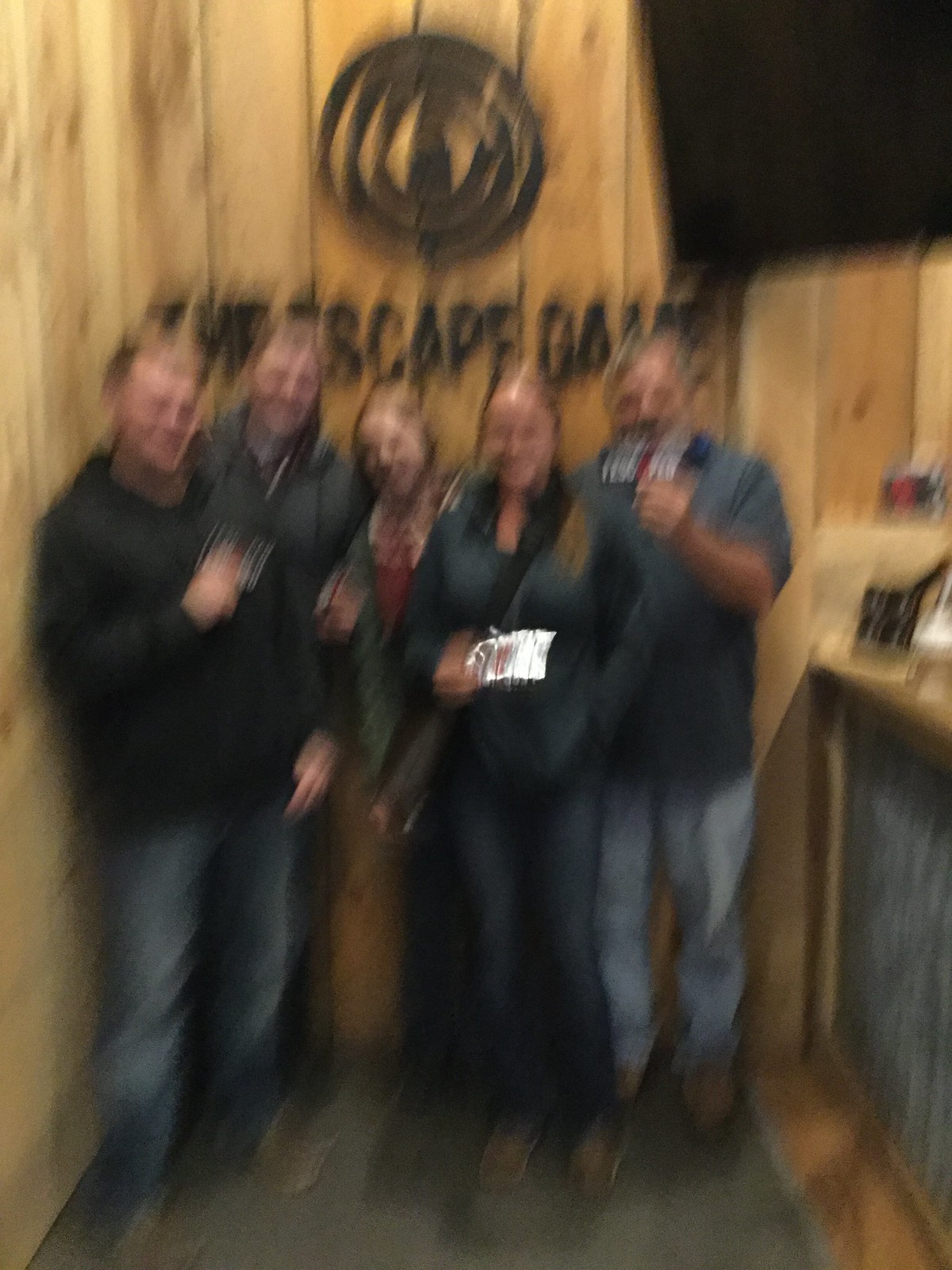In this very blurry color photo, you can see a group of five people standing in what appears to be the reception area of an escape room venue called "The Escape Game." The backdrop features a wood-paneled wall with a black sign that reads "The Escape Game," adorned with a circular logo above it. The group comprises two women in the middle and three men, flanking them on either side, all dressed mainly in dark gray or black tops and blue jeans or dark pants. One woman is distinguishable by her green jacket, while the others wear similar dark attire, including brown shoes. They stand behind a counter, which has a visible black base and various items on top, and they appear to be posing happily, possibly holding an unidentifiable white paper. A TV, currently turned off, is mounted above them, contributing to the overall dark and shadowy ambiance of the scene. The photo also captures part of a black rug on a wooden floor, adding to the establishment's cozy yet modern aesthetic.